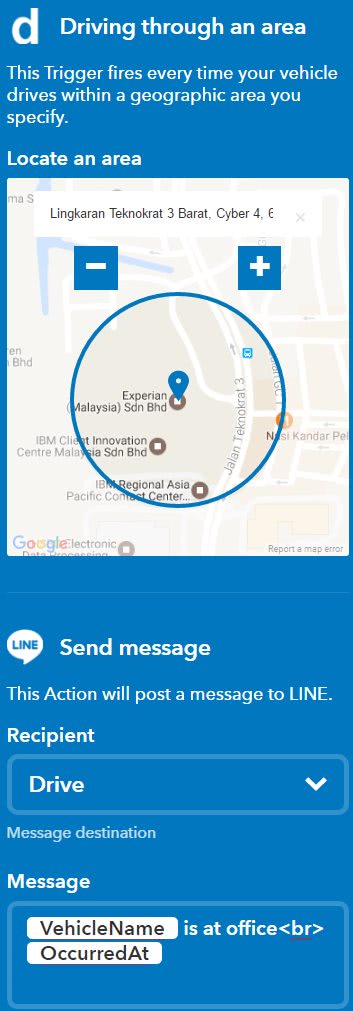Clear and Descriptive Caption:

In this image, a user interface map shows the intricate details of a specified geographic area that triggers an alert whenever a vehicle enters. The central blue circle highlights the activation zone. The map encompasses various labels including "Flink," "Huron," "Technocrat," "Thurber," "Cyber4," "Blue Square," "The Minus," and "Plus." Annotations indicate notable locations such as "Experian," "SDM," "BHT," and the "ABM Client Innovation Center" in Malaysia. At the bottom, blue text signifies an option to send a message via "Line," detailing the vehicle name and destination. The interface prompts that selecting this option will notify the recipient, which is shown as "office, BR, Accuradon." Additionally, borders defining the geographic areas are visible, and the bottom of the map displays the Google logo, signifying the map source. This detailed visualization aids in monitoring and managing vehicular movements within specific zones.